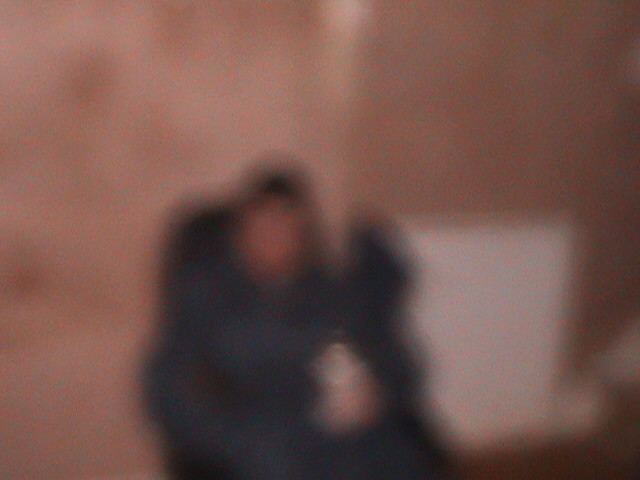The image is a highly blurry color snapshot featuring a man, discernible despite the lack of focus. He is seated in a chair, wearing a black suit and a watch with a reflective, silver finish. His dark hair contrasts with his light skin. The background is a mix of fuzzy, tan, and brown hues, with indistinct shapes suggesting furniture and possibly a small refrigerator or cabinet to the right. There is a hint of a white square that might be a window or another piece of furniture. The overall scene is blurred to the point where finer details meld into vague shapes, but the central figure of the seated man is identifiable.